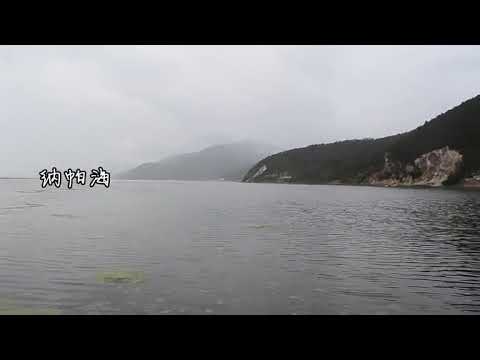The image captures a dramatically overcast day with a dark, almost black body of water that reflects the stark white, cloudy sky. It appears to be a bay, possibly part of an ocean or a large lake. The water seems slightly rippled, and there is some floating vegetation, potentially algae or moss, in the lower left corner. The scene is further framed by two land formations jutting from the right. The nearer one is tree-covered with rocky outlines, while the further one appears mountainous and cloaked in mist or clouds, with some sheer white cliffs visible. The horizon is adorned with four Asian characters, likely Japanese or Chinese, in white with a black outline. The image is bordered by horizontal black strips at the top and bottom, suggesting it may be a screen grab. Despite the cloudy and dark conditions, the landscape's natural beauty is evident, albeit shrouded in the somber tones of the day.